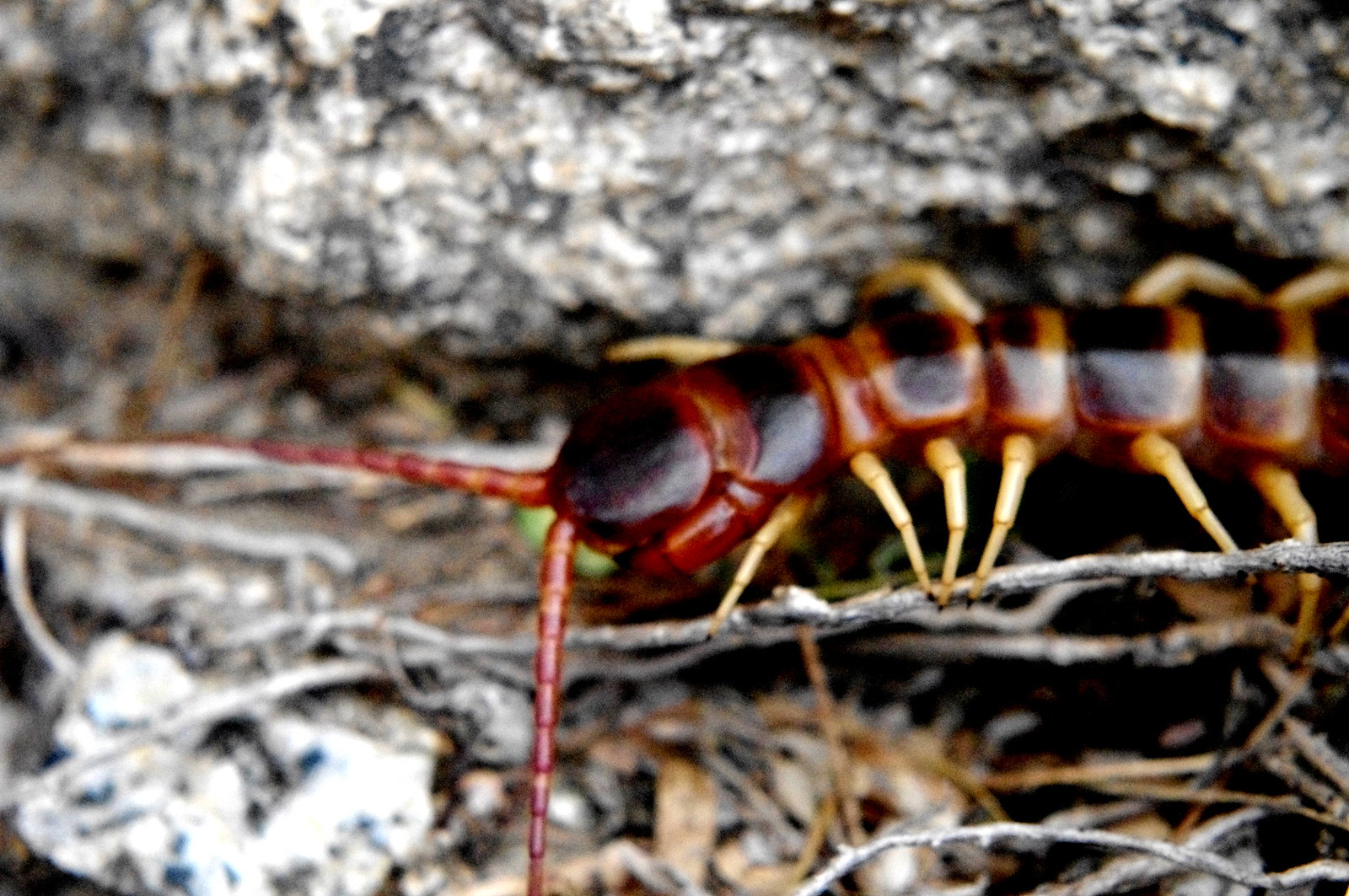The image is a detailed close-up of a centipede situated toward the right center and extending downwards, with its head and segmented antennae pointing towards the bottom left corner. The centipede features strikingly segmented body parts with a dark brown to black central coloration, interspersed with orange to red and light yellow or golden rings around each segment. The legs are off-white to light brown, sharp, and spiky, giving the insect a distinctive appearance as it perches on a thin, silver-like branch. The background showcases a silvery-gray, shiny rock surface that appears as though it had been moistened by rain and dried under the sun. Below the rock, the ground is covered with dirt, leaves, rotting material, and several twigs in brown and gray hues. This detailed natural scene captures the intricate details of the centipede in its rugged outdoor habitat.